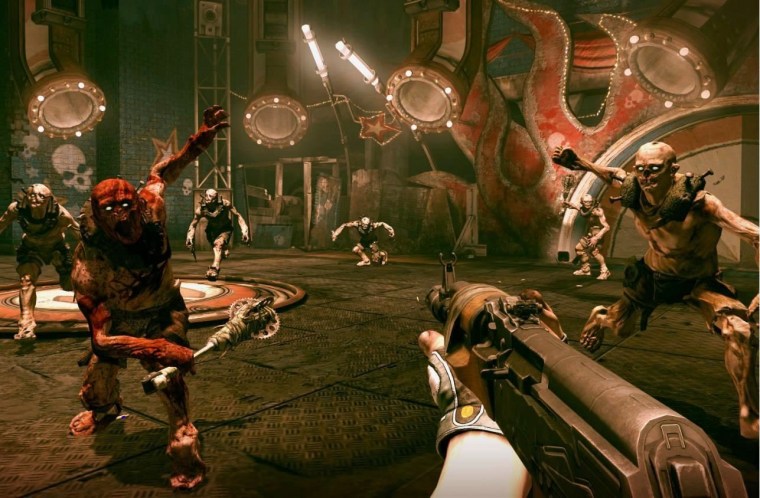This detailed image appears to be a still shot from a video game, showcasing a dystopian or possibly warehouse-like environment. The background features a cinder block wall adorned with numerous paintings and drawings, including small skulls. The floor resembles metal tiles, and there are two large lights overhead that cast an eerie glow on the scene. 

In the foreground, we observe a first-person perspective with a hand gripping a gun. In this chaotic setting, there are five skeletal figures with distinct features. The most prominent figure is on the left side: a red-hued skeleton emanating red light, poised to swing a long weapon with a round blade. The other skeletons trail behind, some adorned with green accessories around their necks and waists, giving them a uniform look akin to armored zombies. Broken pieces of wood litter the area, adding to the sense of desolation and disarray. The entire composition imparts a sense of urgency and impending conflict.